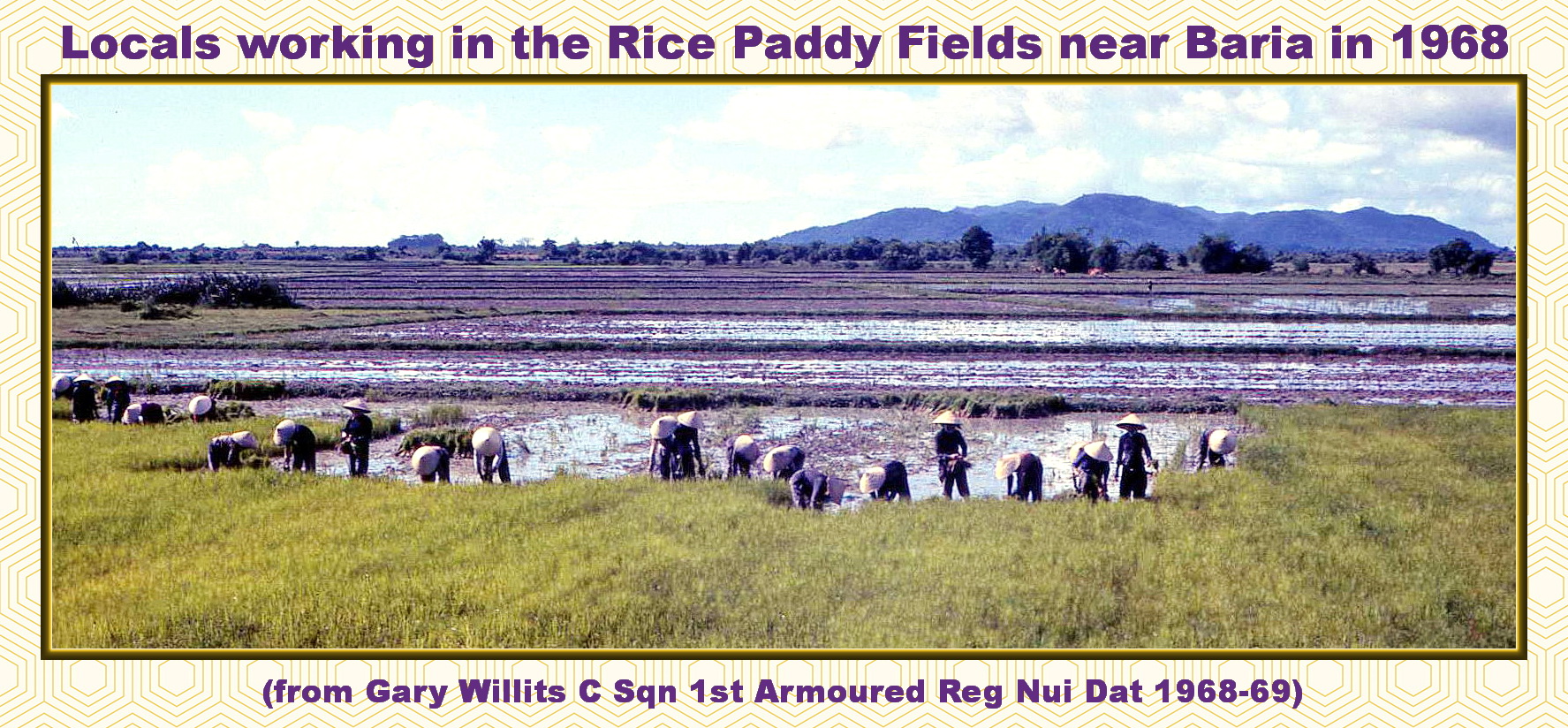This is a color photograph titled "Locals Working in the Rice Paddy Fields Near Baria in 1968." It depicts around 20 people working in lush, flooded rice paddies, characterized by vibrant green grass. The workers are adorned with iconic white, conical hats that are slightly pointed at the top. In the background, a serene mountain range or hill stretches across the horizon, transitioning to dense trees and bushes as the landscape moves forward. The foreground is filled with rows of rice plants awaiting harvest. At the bottom of the image, a caption in parentheses reads, "From Gary Willits C-Squadron First Armored Reg. Nui. 1968-69." The photograph is bordered by a brown frame with a white and tan hexagonal pattern serving as the backdrop. Despite its age, the image offers a vivid glimpse into agricultural life during this period.